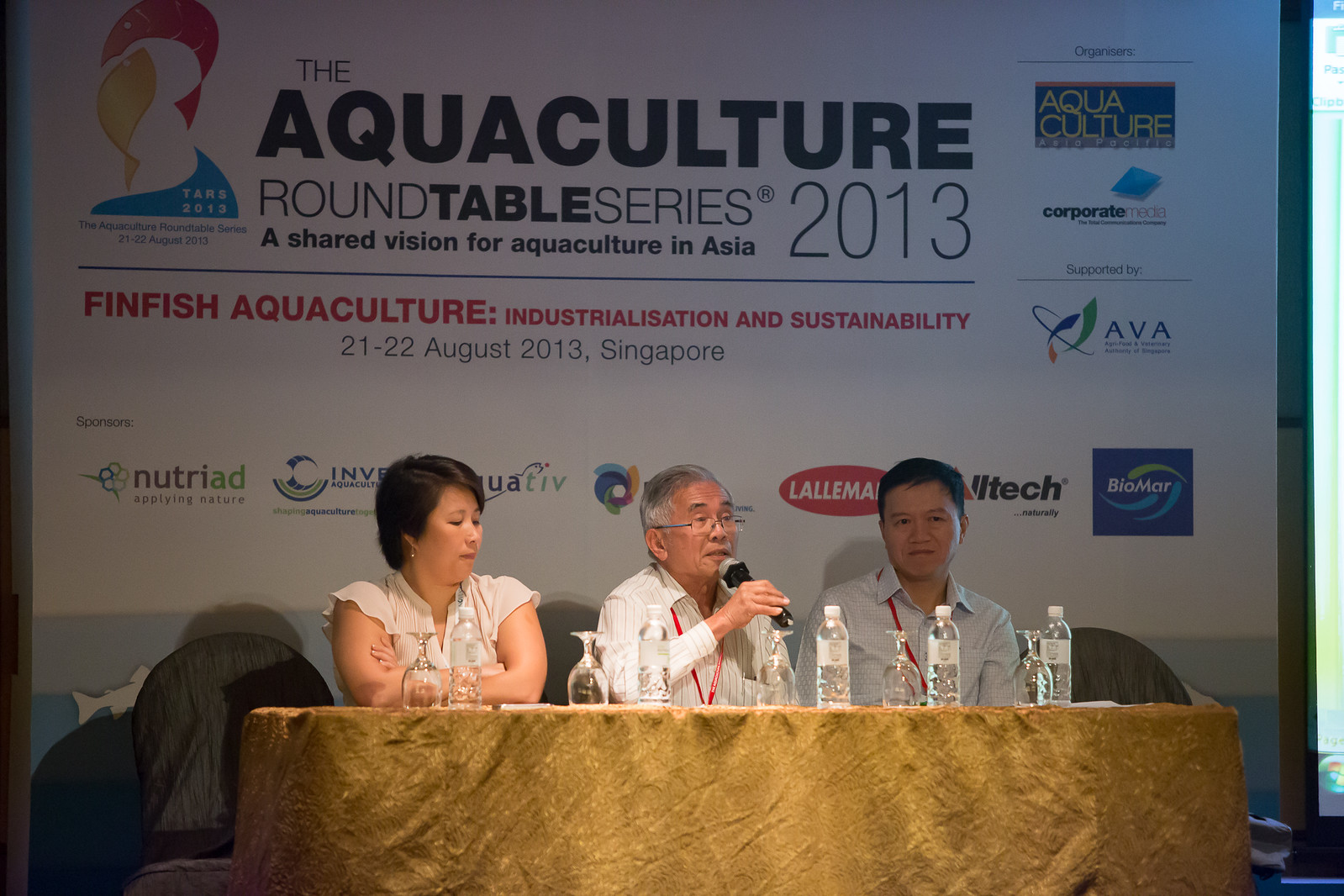In the photograph, three individuals are seated behind a table adorned with a gold tablecloth at what appears to be a convention center. The table hosts an arrangement of five clear water bottles with white caps and labels and five upside-down wine glasses, hinting at a formal event setting. The trio includes a woman to the left with short black hair, wearing a cream-colored blouse, who is looking down towards the center. Seated in the middle is an elderly man, possibly in his 60s, with slicked-back gray hair, glasses, and a white button-up shirt featuring vertical brown stripes, complemented by a lanyard. On the right is a younger Asian man with black hair, a red lanyard, and a button-up collared shirt in a bluish-gray hue.

The backdrop features a prominent white sign announcing "The Aquaculture Roundtable Series 2013: A Shared Vision for Aquaculture in Asia," with "FinFish Aquaculture Industrialization and Sustainability" highlighted in red text. Additionally, it specifies the dates "21-22 August 2013, Singapore." The sign is adorned with various logos, including "AVA" and "Biomar" in a blue square, alongside numerous other partially obscured logos presumably representing event sponsors. The overall atmosphere suggests a formal discussion or presentation, potentially addressing an audience on topics related to aquaculture.